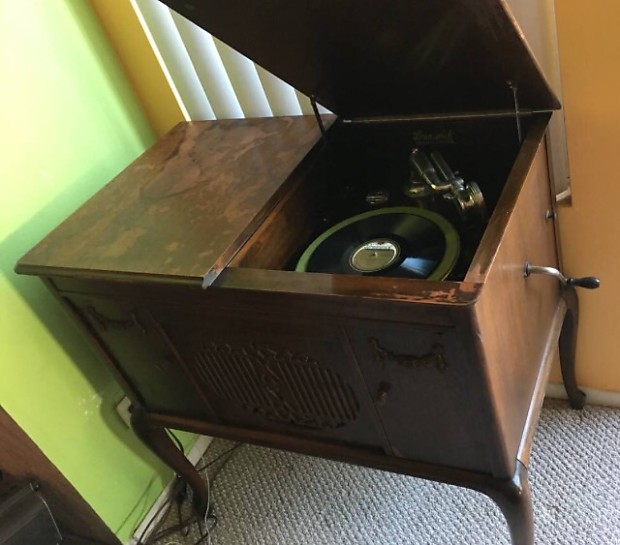The photograph captures a vintage wooden music box, standing elegantly upright on four curved legs atop a gray carpet. The music box is dark brown in color and features two lids at the top; the right lid is open, revealing a circular black vinyl disc mechanism, while the left lid remains closed. Attached to the side of the box is a chrome crank handle with a black knob. The background includes a green-painted wall on the left side, with an orange-painted wall directly behind the music box, complemented by white curtains. The overall setting has a furniture-style atmosphere, combining elements of nostalgia and functionality.